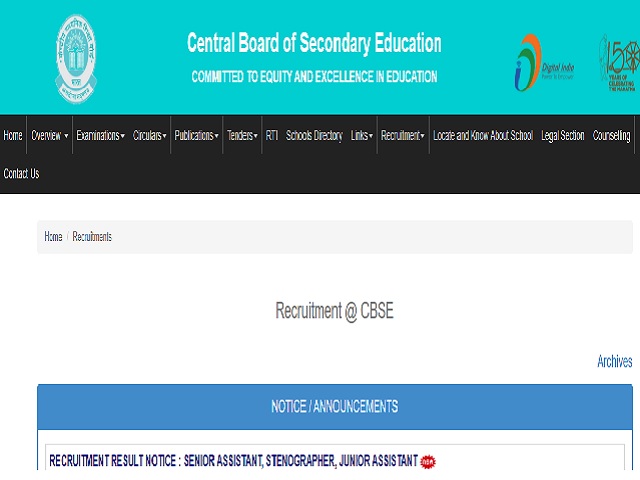The image features a webpage header set against a turquoise, teal-colored background. At the top, the text "Central Board of Secondary Education" is prominently displayed, followed by the tagline, "Committed to Equity and Excellence in Education." The header also includes several symbols: one on the left and two on the right, although they are too blurry to identify distinctly.

Beneath the header is a black navigation bar with a series of drop-down menus and clickable links. These include options such as Home, Overview, Examination, Circulars, Publications, Tenders, RTI, School Directory, Links, Recruitment, Locate and Know About School, Legal Section, Counseling, and Contact Us.

Following the navigation bar is a light gray box containing breadcrumb links that read Home > Recruitment. The subsequent section is titled "Recruitment at CBSE" and includes a blue hyperlink labeled "Archives" as well as a blue button labeled "Notice Announcements." Below these are specific recruitment notices listing positions such as Senior Assistant, Stenographer, and Junior Assistant.